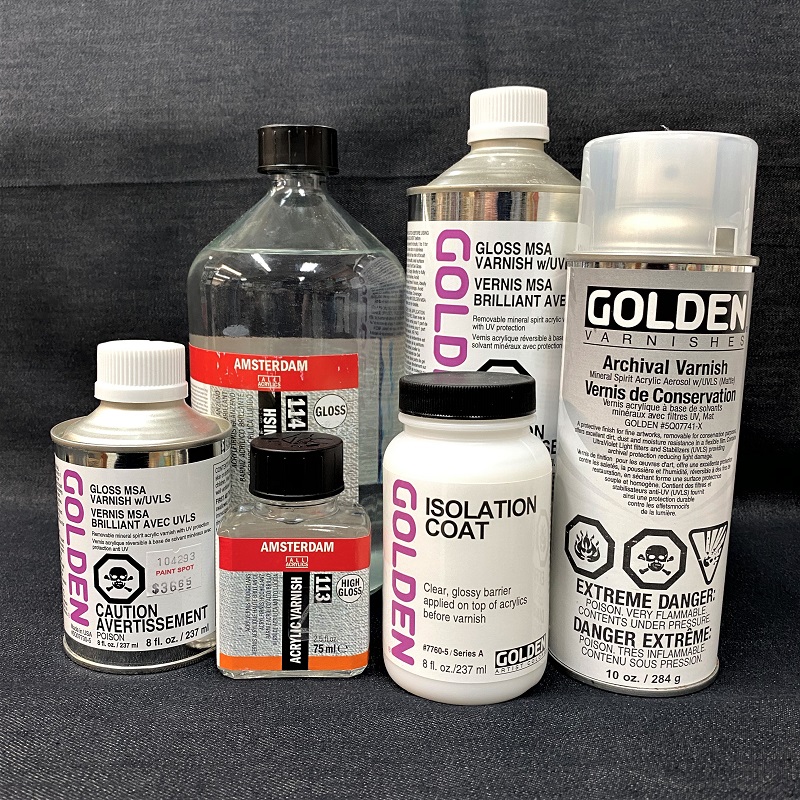The photograph showcases an assortment of six painting-related products displayed against a solid black background. These items include varnishes and isolation coats from various brands like Golden and Amsterdam. The containers are diverse in material and shape, featuring aluminum cans, glass bottles, and one plastic bottle. Prominent in the foreground is a white plastic bottle with a black cap labeled "Golden Isolation Coat" in purple and black text. Alongside, there's a metallic can marked with "Golden Gloss MSA Varnish," caution labels, and an "8 fluid ounces" specification. Another clear bottle from Amsterdam reads "High Gloss 113" and "75 milliliters." A larger grey spray can labeled "Archival Varnish" with various warning texts is also featured. Across the composition, the products display vibrant colors such as orangish red, gold, silver, black, white, purple, and grey. All bottles and cans stand upright in a vertical rectangle format, with the taller items positioned at the back and smaller ones at the front, making the different sizes and branding evident. The image, likely taken for product display purposes, emphasizes the clarity of labeling and the variety of varnishes available.